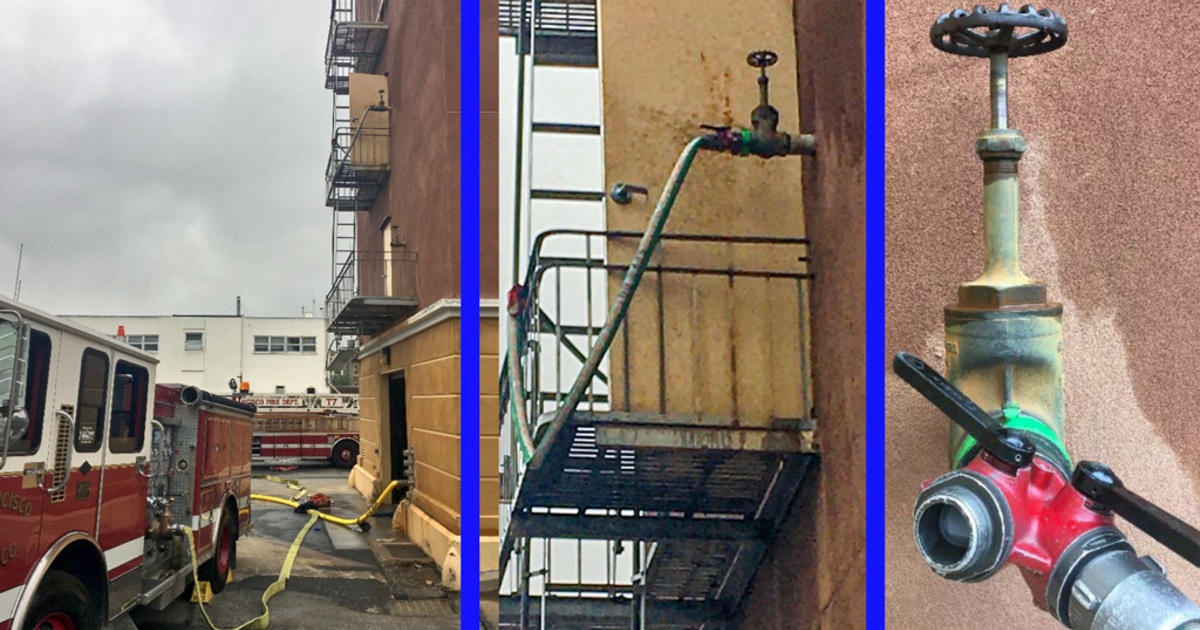The image depicts the exterior of a multi-level apartment building in an urban setting, detailed in three horizontally arranged frames separated by blue lines. The building showcases a yellow brick base with a red stucco upper half, and features multiple metal fire escape staircases. In the left frame, two firetrucks are seen parked on the pavement, each with hoses hooked up to a fire hydrant, indicating a recent or ongoing emergency response. The middle frame zooms in on a landing area between two floors of the apartment, highlighting an open door with a hose connected to a faucet on the building's exterior. The right frame offers a close-up view of this connection, detailing the hose and the valve attached to the wall.